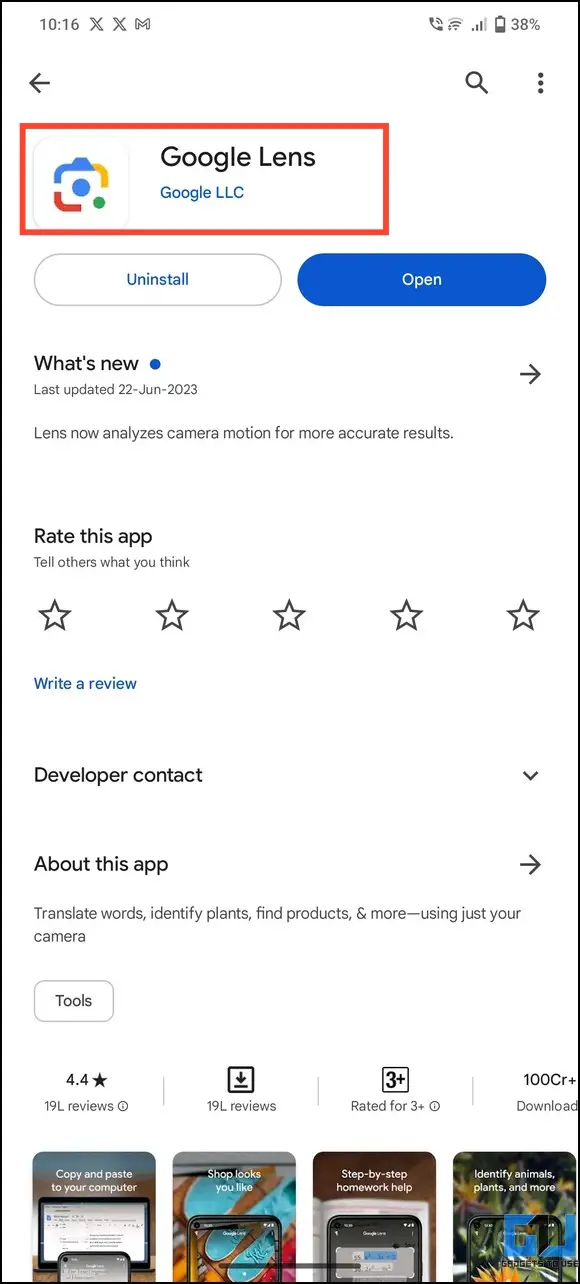The image showcases the Google Lens app page on the Play Store, specifically on an Android device. Dominating the center of the screen is the Google Lens logo, which depicts a stylized camera outline composed of Google's signature colors. The page indicates that the app is already installed, as evidenced by the presence of both "Uninstall" and "Open" buttons.

Directly below these controls is the "What's New?" section. The app's last update was on June 22, 2023, and the latest improvement includes an enhanced ability to analyze camera motion for more accurate results.

Users are prompted with the option to rate the app, and there is a link to write a review. Additionally, there is an expandable "Developer contact" section for further details.

The "About this app" section offers a brief description of Google Lens' capabilities, which include translating words, identifying plants, finding products, and more through the use of the device's camera. Beneath this description are a series of images demonstrating various outdoor uses of the app, although these images are partially cut off in the view.

The app has a rating of 4.4 out of 5 stars, with what seems to be a discrepancy in the reviews and downloads data. The display shows "1,000 reviews," but there is also a mention of "19 L reviews," where "L" might be intended to represent a Roman numeral. However, this seems unclear. The total number of downloads reads as "19,000."

Overall, the image provides a comprehensive look at the Google Lens app's Play Store page, highlighting its features, current user feedback, and some usage examples.